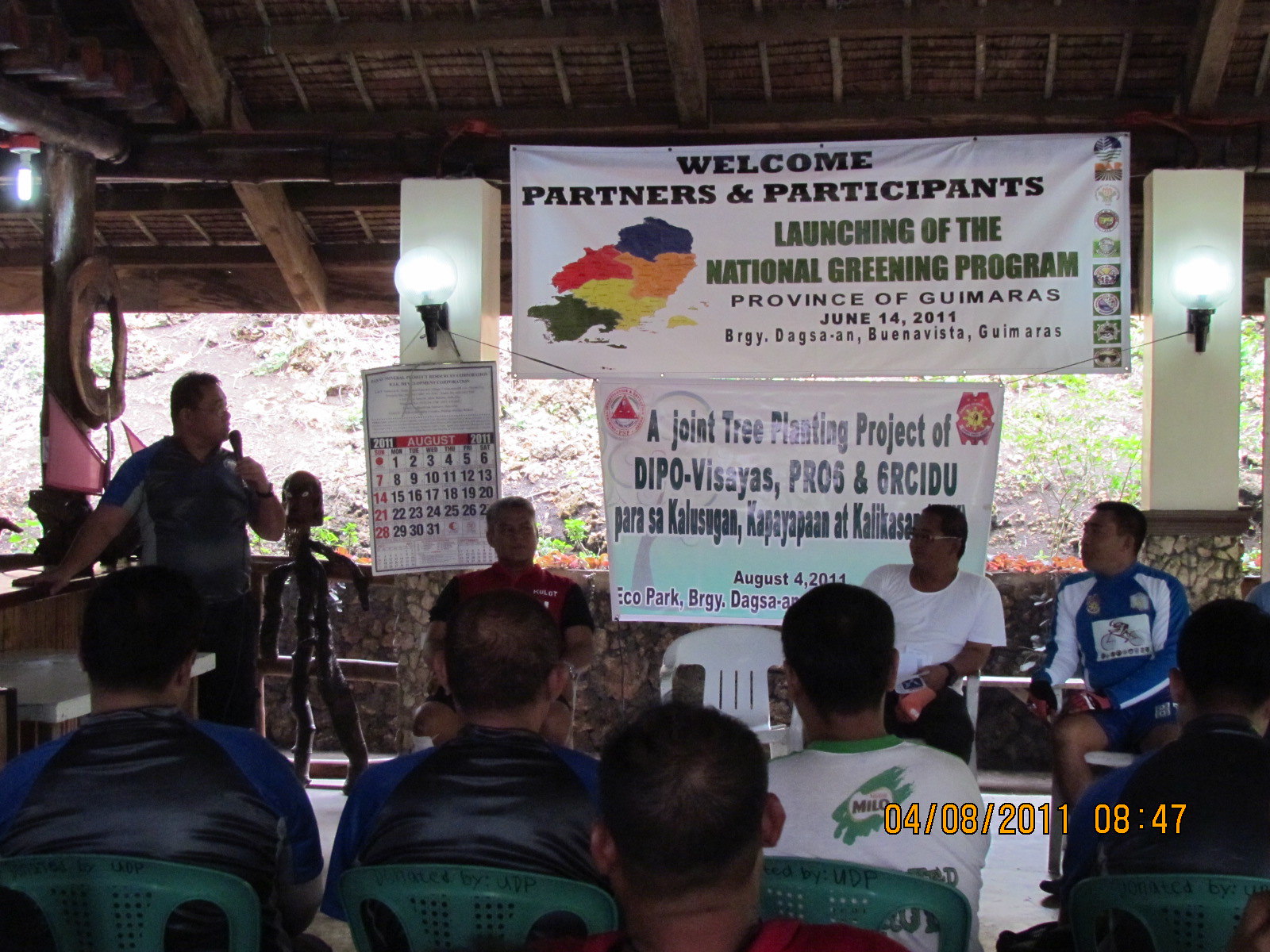The photograph captures a lively gathering at an indoor-outdoor venue with no walls, allowing views of the surrounding trees. The event features multiple attendees seated in green and white plastic chairs, some sitting on a stage while others occupy spaces in the foreground and throughout the audience. Prominently, a man in a blue short-sleeved shirt stands to the left, speaking into a microphone. Above the stage hangs a large, plastic banner with the text: "Welcome partners and participants. Launching of the National Greening Program. Province of Guimaras, June 14th, 2011." Beneath this message, another banner reads: "A joint tree planting project of DIPOVISAYAS, PRO and GRCIDU," followed by the date "August 4th, 2011." The venue is characterized by its rustic, hand-hewn wooden beams, and to the left of the stage, a calendar shows the date "August 2011." The serene setting and attentive audience contribute to the event's focused atmosphere.